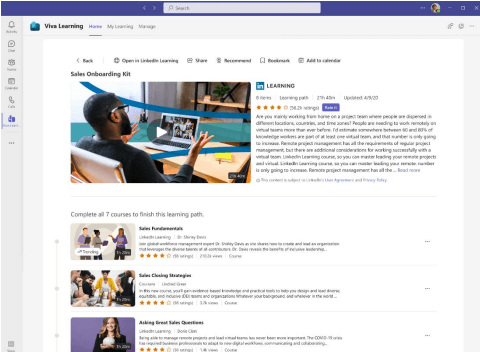This screenshot, taken from an electronic device resembling a 13-inch MacBook, features the interface of Viva Learning. The interface displays a neatly organized layout despite the small size of the screenshot. The header includes navigation options such as "My Learning," "Home," and "Manage," alongside various icons including an avatar, a bell, a badge, and several indicators. There's also a home button and an up button, all set against a gray background.

At the very top, we have a search box and a tiny "X" in the upper right corner, accompanied by three dots for additional options. The upper right corner also includes a small avatar set against a blue background.

Central to the screenshot is the "Sales Onboarding Kit" section. This includes an image of an individual seated at a desk with an open laptop, underlining the learning content being offered. The prominent section heading reads "Learning" and is accompanied by a rating system, showing four out of five stars.

Beneath the heading, there are various segments detailing the progression path, such as "Complete all seven courses to finish this learning path." Specific course names like "Sales Professionals," "Sales Checking Strategies," and "Asking Sales Questions" are visible, each featuring images representing conversational sales scenarios.

Despite the small size and some text being almost unreadable, the overall structure and key elements like the sales onboarding kit and learning path content are discernible, suggesting a comprehensive and user-friendly learning platform.